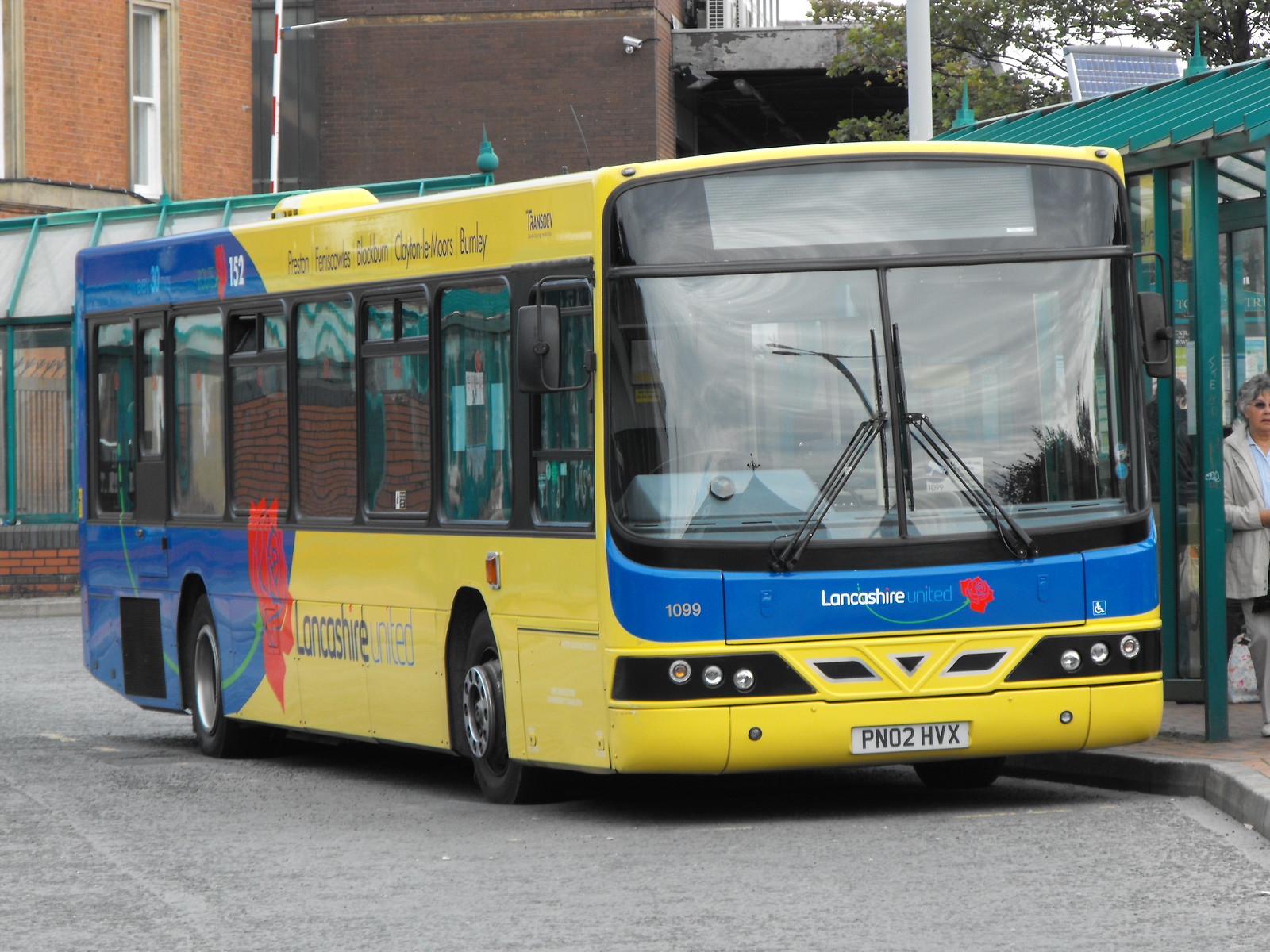This image depicts a front-side view of a large yellow and blue bus with a sizeable windshield and windshield wipers, prominently labeled "Lancashire United" with the license plate "PN02HBX." The bus is stationary at a bus stop, with a lady waiting in the light blue-green bus stop shelter to the right. Surrounding the scene, there are brick buildings—some light brown and dark brown—in the background, and green trees at the top right. Below the bus, the road appears gray. A security camera is mounted on one of the buildings above the bus. The bus also features additional colors with accents of red, green, and white from the license plate.